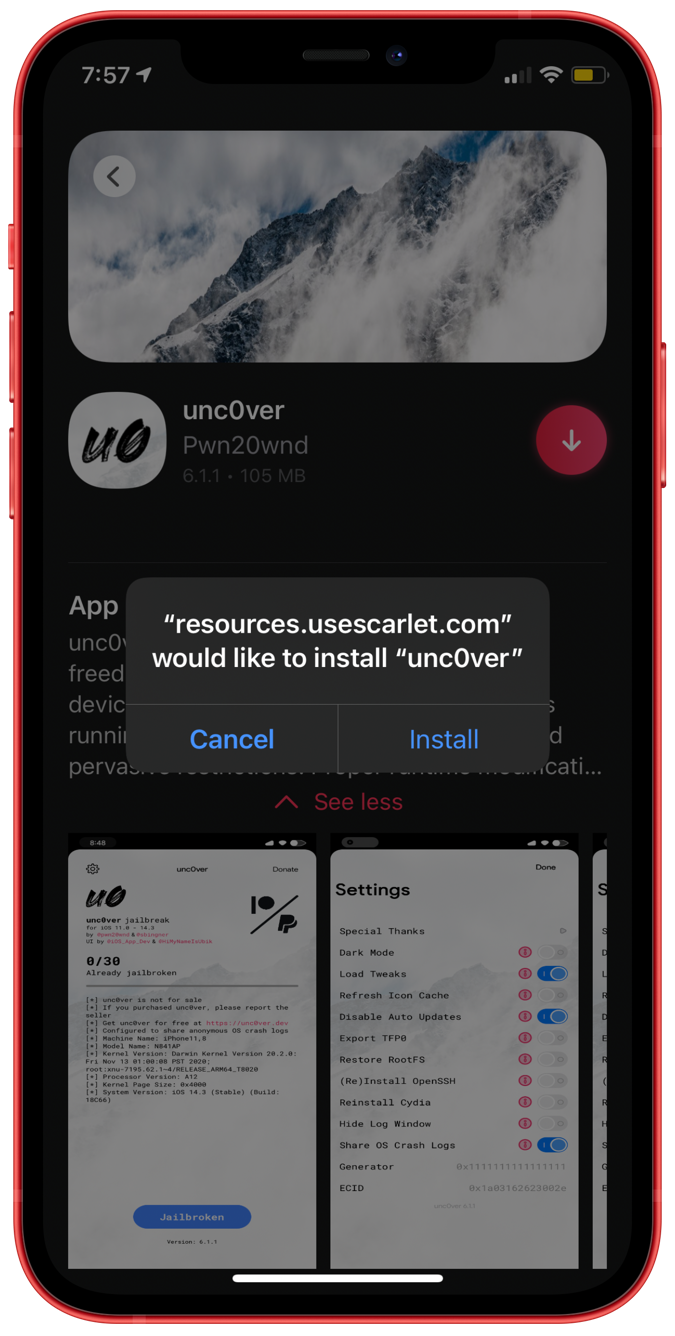The image is a vertical rectangle, prominently displaying a smartphone outlined by a thin orange border. On the left side of the phone, multiple buttons are visible, whereas the right side features a single button, suggesting that the device is likely an iPhone.

At the top-left corner of the screen, "7:57" is shown in white text accompanied by an arrow pointing to the upper right. Moving across the top, there is a signal strength indicator showing "2 of 4" bars, followed by a Wi-Fi icon with three bars, and a battery indicator that appears to be approximately half-charged.

Below these indicators, the main display shows an image of a mountain landscape partially obscured by clouds. An arrow pointing to the left is visible at the top of this image. Beneath this, a white box contains black text with the letters "UO," and to its right, the text "uncover PWN 20 WND" can be seen. Additionally, there is a red circle featuring a white downward-pointing arrow on the right side.

Overlaying this background content is a pop-up window with the message: "resources.uscarlet.com would like to install uncover," followed by two options: "Cancel" or "Install."